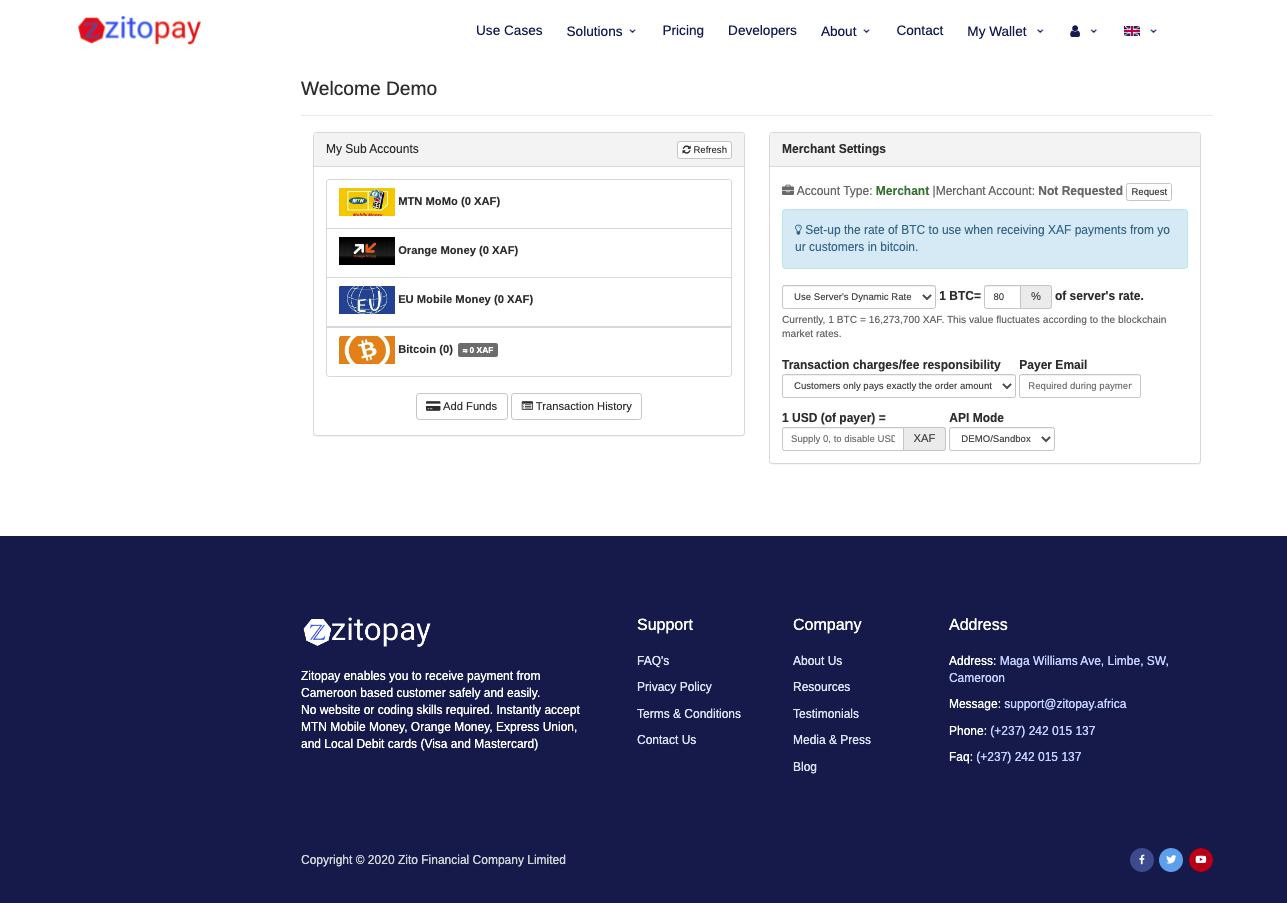Certainly! Here is a detailed and cleaned-up caption:

---

The webpage for Zetopay showcases a clean and organized interface on a white background. At the top, the brand name “Zetopay” is prominently displayed, with "Zeto" in blue and "pay" in red. In front of this name sits an icon: a blue "Z" encased in a red hexagon. Across the same line, starting from the middle of the page and moving right, there are several menu items and dropdown options: "Use Cases," "Solutions" (with a dropdown), "Pricing," "Developers," "About" (with a dropdown), "Contact," "My Wallet" (with a dropdown), a profile icon (with a dropdown), and a British flag (with a dropdown).

Beneath this navigation bar, a greeting reads "Welcome Demo," followed by links to "My Sub Accounts" and a refresh button. Further below is a list of sub-account balances:

- MTN Momo (0 XAF)
- Orange Money (0 XAF)
- EU Mobile Money (0 XAF)
- Bitcoin (0 = 0 XAF)

To the right side, a section titled "Merchant Settings" indicates the account type as “Merchant” in green. It also notes a “Merchant Account” status as "Not Requested" with a button to "Request." Below this section, within a blue background, instructions read: "Set up the rate of BTC to use when receiving XAF payments from your customers in Bitcoin."

---

This caption comprehensively describes the key elements and layout of the Zetopay webpage.